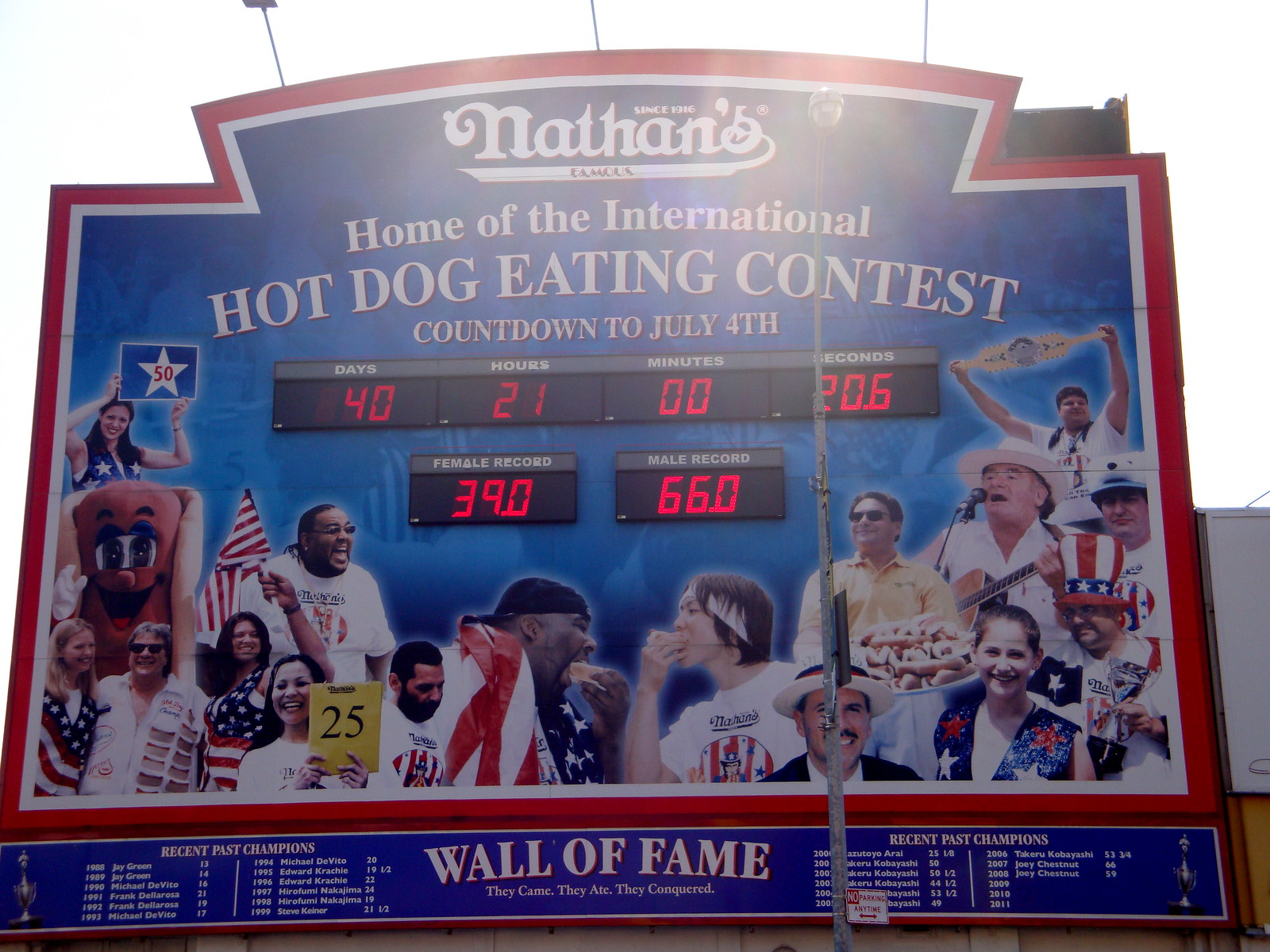The image showcases a rectangular billboard for Nathan's Famous, prominently displaying a red and white border. At the top of the sign, "Nathan's Famous" is written in bold white font. Directly below, in all caps, it reads "Home of the International Hot Dog Eating Contest." Beneath this, another line in smaller capital letters states "Countdown to July 4th." The countdown timer is digitally presented in glowing red numbers indicating 40 days, 21 hours, 0 minutes, and approximately 20.6 seconds remaining. The sign also highlights records for the contest, listing the female record at 39 hot dogs and the male record at 66 hot dogs.

In the bottom portion of the billboard, there is a vibrant collage of images. This includes participants and spectators draped in American flags, individuals holding hot dogs, a plate of hot dogs, a guitar player, and a person triumphantly raising a championship belt. Further down, a blue footer labeled "Wall of Fame" with white text underneath showcases columns of names, presumably recent and past champions. The layout suggests that these might be grouped by gender, with separate sections for male and female champions.